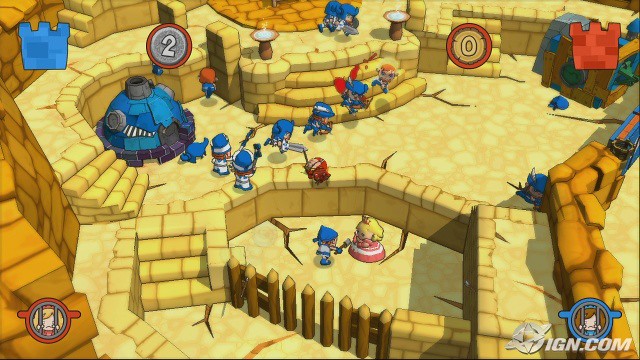The image depicts a scene from the video game "Fat Princess," set in a desert-like medieval environment characterized by tan or golden stone blocks and structures. The central focus is a battlefield with castle-like elements, including turrets made from dark brown stone walls and spiked wooden fences for protection. In the bottom center, a princess adorned in a pink and white gown with blonde hair and a pink crown appears to be interacting or fighting with blue-capped soldiers. Blood is scattered on the tan stone steps leading up to different levels. 

Prominently positioned is a large, rotund figure in blue attire with a black bottom, seated on a rounded throne, potentially the commander orchestrating events. To his left is a blue and gray dome-like machine, possibly coal-powered, with the number two displayed overhead. The image also shows various small soldiers dressed in blue and white, part of the red versus blue teams, indicated by the red "0" near a red castle and a blue castle symbol. Finally, the watermark "IGN.com" is visible in the bottom right corner.